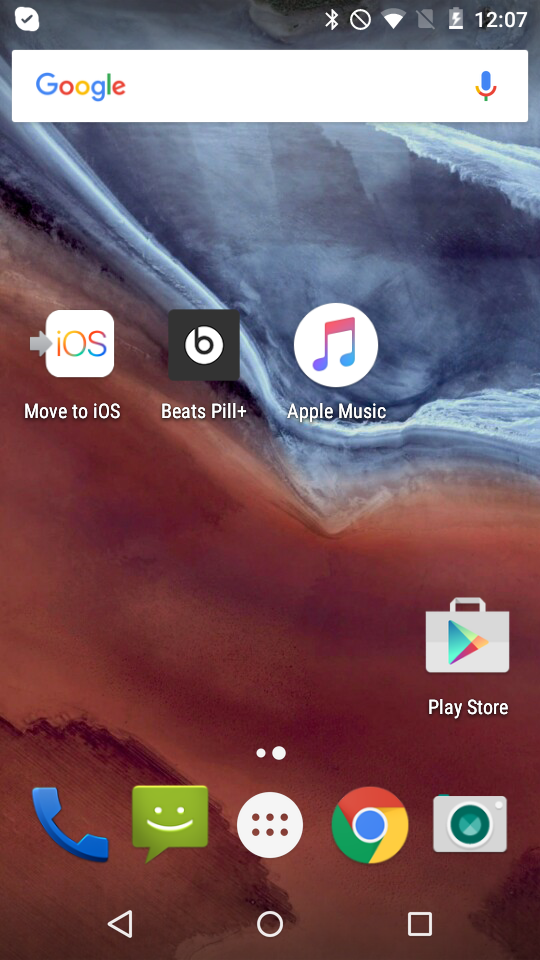In this image, we are viewing a screenshot from a cell phone. At the upper left corner, there is a checkmark inside a white oval shape, and to the right of it, the text reads "Wi-Fi 1207." Below this, there is a large white search bar with the word "Google" on the left and a microphone icon on the right. The background of the phone screen features an abstract design in shades of blue, rust, brown, and gray. 

Several app icons are neatly arranged in a row starting from the left. The first icon is for the "Move to iOS" app, indicated by a gray arrow pointing to the left and the text "iOS" below it. To the right of this is a black box with a white donut shape and the letter "B" inside it, representing the "Beats Pill" app. Next to it is a white circle with a music note icon, signifying the "Apple Music" app. Following this is the "Play Store" icon.

Additionally, across the bottom of the screen, there are four more icons: the telephone app, the messaging app, Google Chrome, and the camera app.